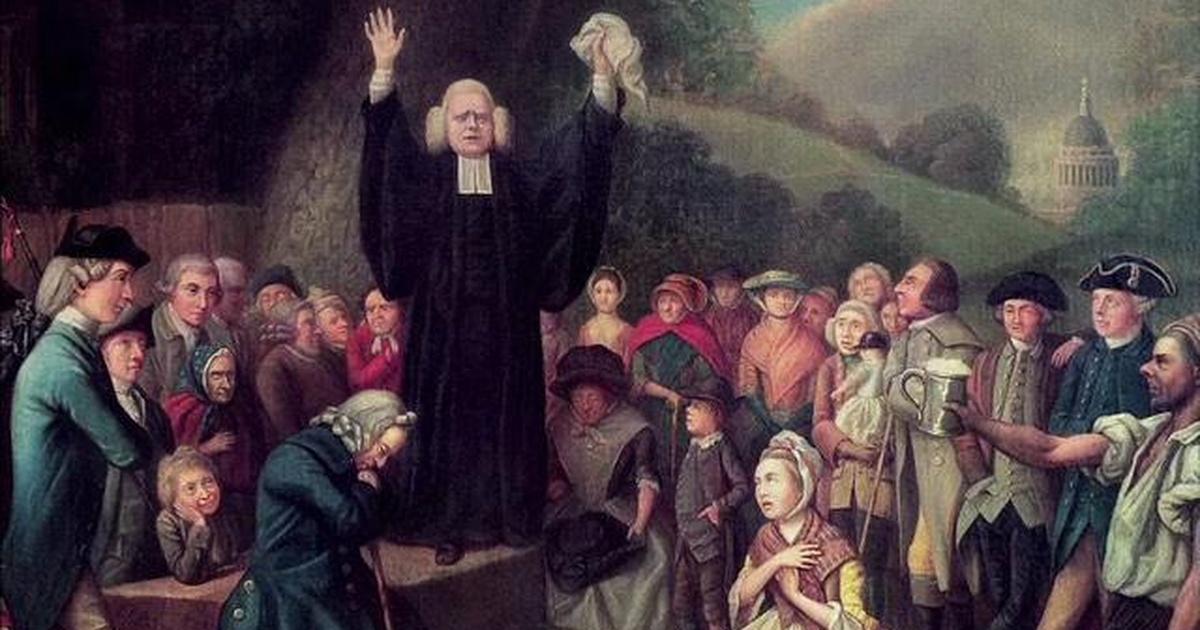This historic painting, rich in vibrant colors and natural light, captures a crowd gathered outdoors, likely in the late 18th or early 19th century. The scene is dominated by a throng of men, women, and a few children, all dressed in period attire including frock coats, three-cornered hats, multi-buttoned coats, full-length dresses with corsets, and bonnets. Some men wear powdered wigs. The crowd is intently listening to a man standing on a wooden box or pedestal, dressed in black robes with a white collar reminiscent of a Roman priest or judge. His gray or white hair complements the dramatic scene as he holds a wig in his left hand and raises his right hand, likely preaching or giving a speech. In the upper right of the painting, the domed roof and pillars of a Capitol-like building are visible, set against a backdrop of green hills, trees, and clouds.